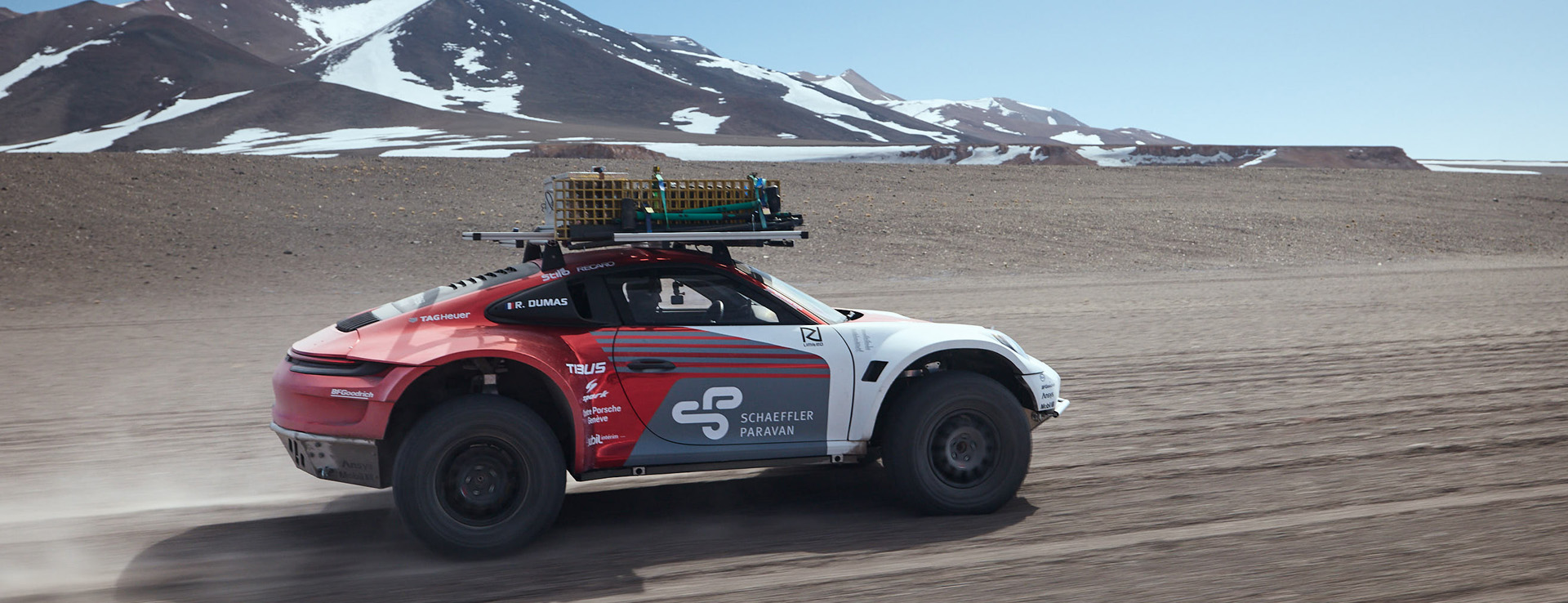In the photograph, a richly detailed scene unfolds under a clear blue sky. Centered to the left, a dynamic truck is captured in motion as it drives through a sandy desert area, evidenced by the dust kicking up from its large, rugged tires. The truck is strikingly painted with a gradient of white at the front, transitioning through gray in the middle to a bold red towards the rear, prominently on the side passenger door. This door features the words "Schaefer Paravan" in white, accompanied by a logo resembling a merged "P" and "S." Additional inscriptions, though partially obscured, include "T-Bus" near the top. 

Above the truck, a metal roof rack holds a complex device, possibly for scientific measurements. The silhouette of the driver is faintly visible through the window. In the backdrop, a majestic black mountain, dusted with snow, rises from the left and extends towards the middle-right, complementing the arid foreground with its stark contrast. The entire scene pulsates with the feel of outdoor adventure and scientific exploration, captured crisply during daylight.